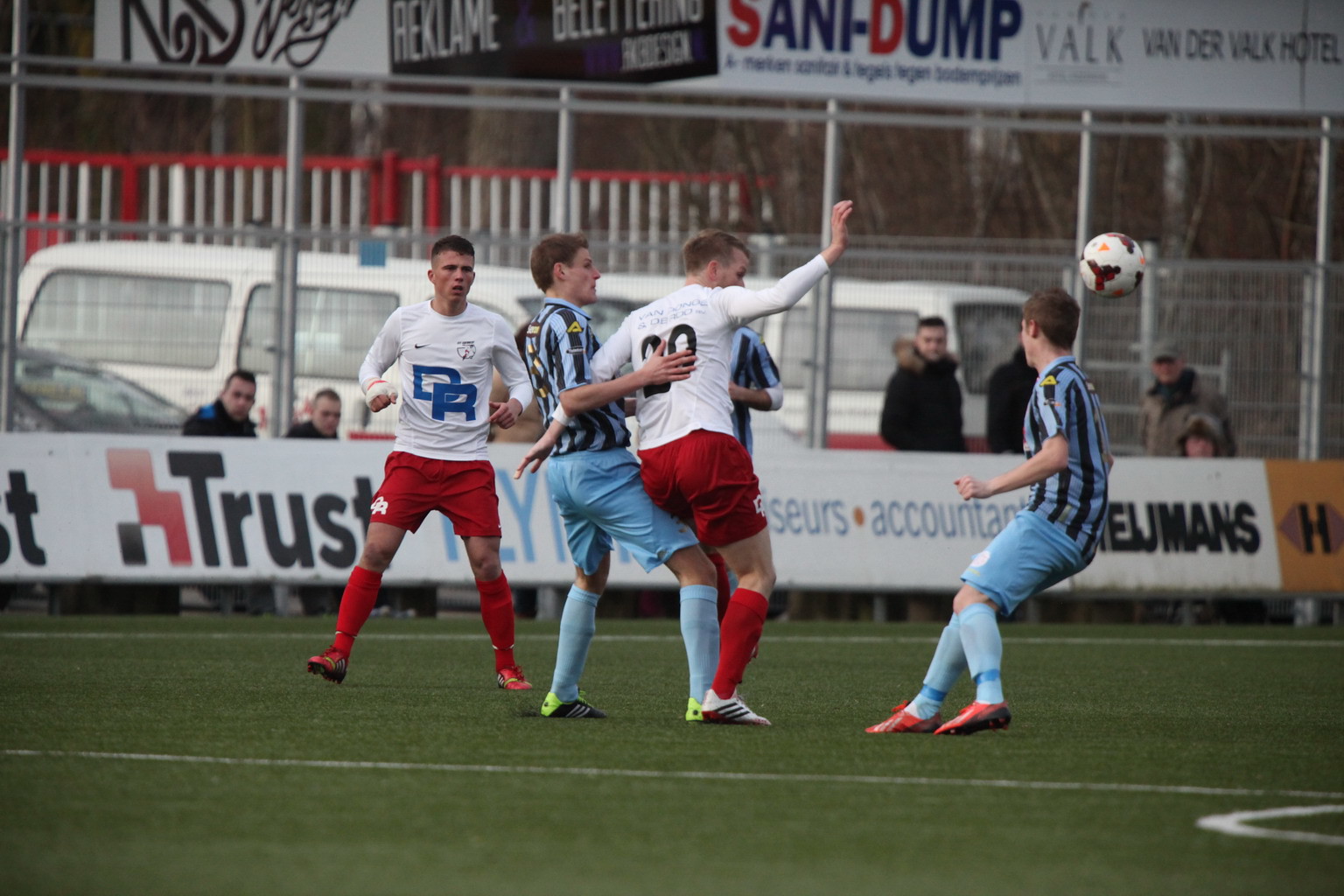The photograph captures an intense moment of an outdoor soccer match, showcasing five players mid-action on a vibrant green turf field. Two players don white long-sleeved jerseys paired with red shorts and socks, while the other three sport light blue and black striped jerseys with matching shorts and socks. The soccer ball, a blur of white, black, yellow, and a hint of purple, is suspended in the air. Surrounding the field is a barricade wall adorned with sponsor logos, prominently featuring the word "TRUST." Above the viewing area sits a banner bearing additional sponsor logos. Behind the barricade, a tall chain link fence separates the field from spectators, who gather to watch the game. In the distance, beyond the fence, a parking lot filled with cars and vans is visible, completing the bustling scene of this spirited soccer match.